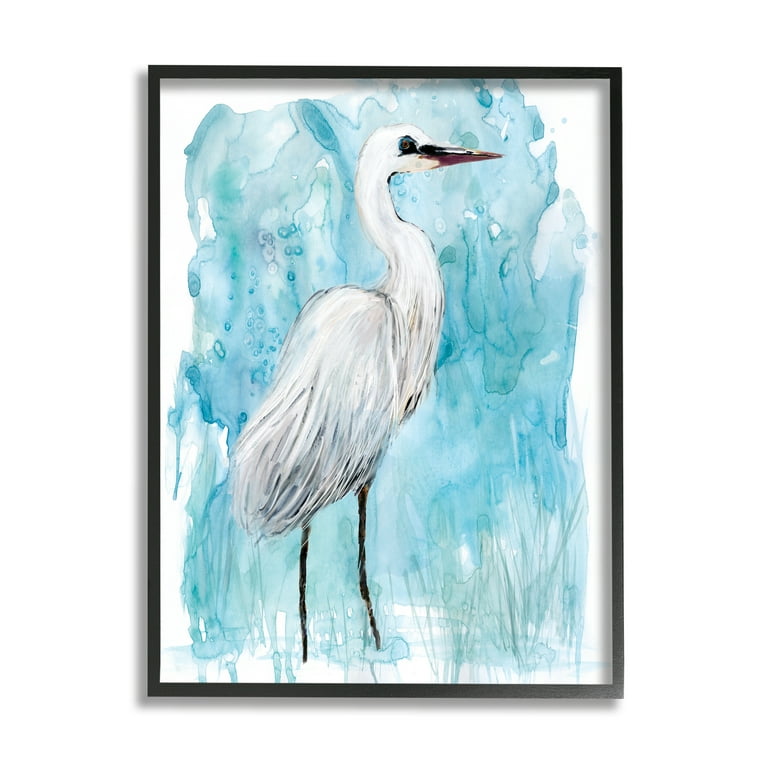The painting depicts a side view of a white crane standing against a predominantly blue watercolor background, which simulates a watery environment. The crane, with its white feathers, long black legs, striking black beak, and prominent black eye, is positioned to face the right. The lower part of the image features green stripes and a very light green watercolor suggesting grass. This artwork, characterized by its watercolor technique, is framed with a narrow black border.